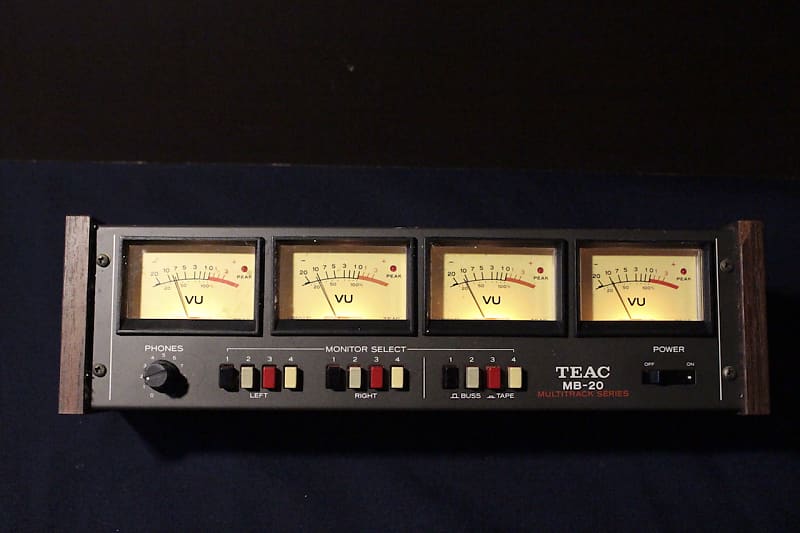The photograph features a vintage-looking, nearly rectangular metallic device in a dark green color. The front panel is flanked by wood panels on the left and right sides. At the top of the device are four yellow meters, each labeled with "V.U." Below these meters, there are various switches and buttons in a pattern of black, red, and cream. On the left side, there's a dial labeled "Phones." Above the buttons, the words "Monitor Select" are visible. On the right side is the power button. The front of the device prominently displays the text "TEAC MB20 Multitrack Series," with "TEAC" in white capital letters and the series name in red. The background of the image is a plain black, with a dark blue surface partially visible behind the device.